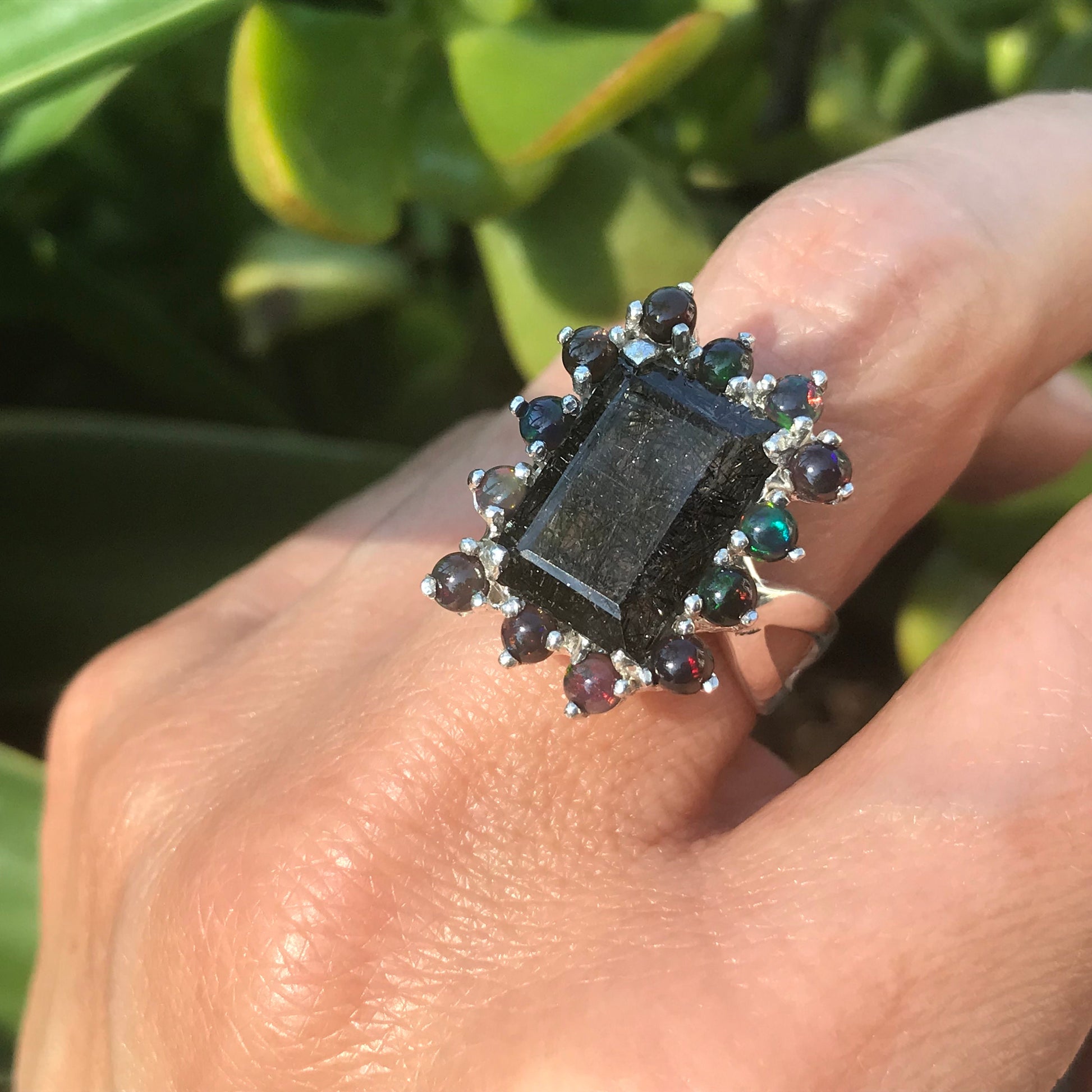This detailed, close-up, color photograph captures a woman's hand modeling an ornate signet-style ring on her index finger, prominently centered in the image. The ring features a substantial rectangular tourmaline stone, greenish-gray with striping, encased in a silver setting with intricate bezel carvings on all four sides, aligning with the elongated shape of the finger. Surrounding the central stone are 13 smaller, round stones or jewels, secured with silver pins, exhibiting a variety of colors including greenish-blue, rose, and gold hues. The band of the ring, also silver, is designed with two open sections, adding to its intricate detailing. The hand, positioned to show the knuckle of the index finger and partial views of the thumb and forefinger, stands out against a slightly blurred background of green foliage, likely from a jade or succulent plant, enhancing the realistic and representational photographic style. The central tourmaline stone appears aged, lending a darker, almost black hue and lacks sparkle, suggesting that it is old or potentially unclean.